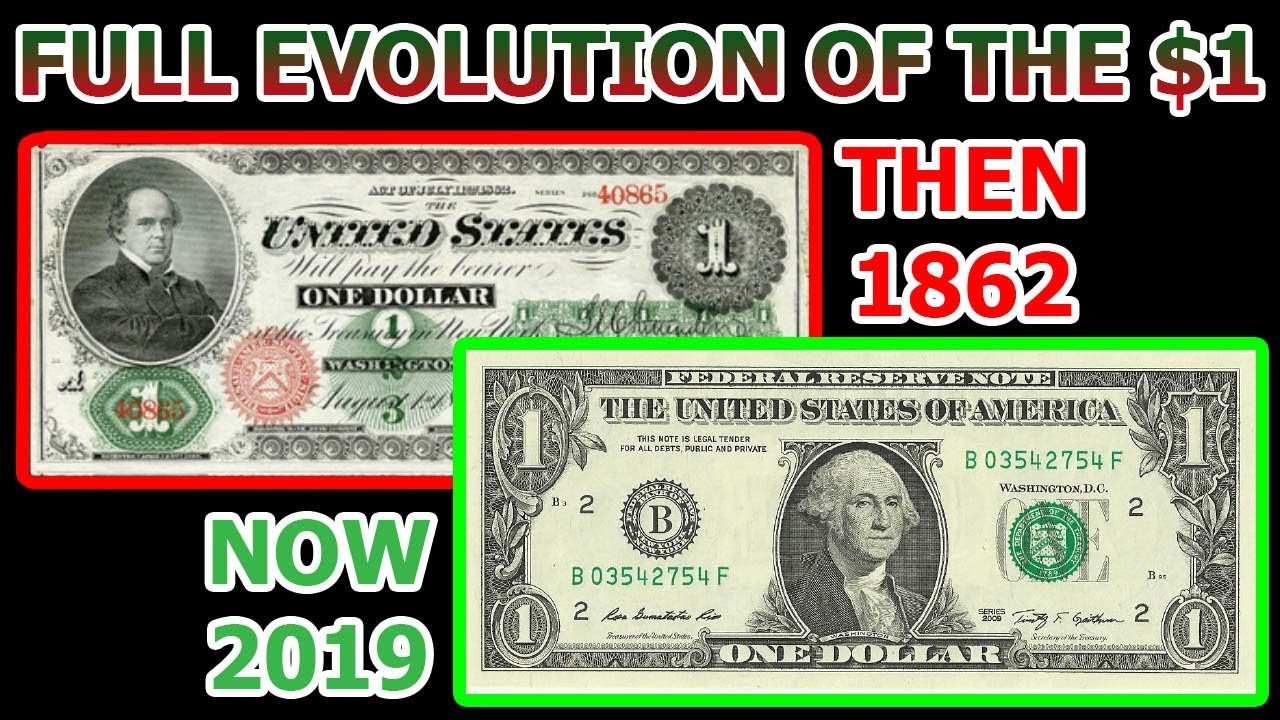The photographic image features a black background with the text "Full Evolution of the $1" at the top, rendered in a gradient of green and red with a white outline. This visually striking graphic serves as a comparison between two different U.S. one-dollar bills from disparate years, 1862 and 2019.

In the upper left section, bordered in red, the outdated dollar from 1862 is displayed. This bill, printed with black ink on a white background, includes intricate details: a smaller portrait of a man (appearing to be a historical figure) in the top left corner, the unique identifying number 40865 in both the top right and bottom left corners, and the explicit text "The United States will pay the bearer one dollar at the treasury of New York, Washington, August 3rd." The number "1" is featured prominently in the top right corner. The caption for this section reads, "Then 1862."

In the bottom right section, bordered in green, the image reveals the modern one-dollar bill from 2019. This bill is easily recognizable with its green coloring and the prominent portrait of George Washington at the center. It is labeled "Federal Reserve Note" and declares, "This note is legal tender for all debts, public and private." The dollar bill features the serial number "B03542754F" displayed in the top right corner, replicating the serial number on the bottom left corner. The number "1" appears in all four corners of the bill, consistent with its current design. The caption here reads, "Now 2019."

This image compellingly shows the evolution of the U.S. one-dollar bill over time, capturing the distinct changes in its design and presentation.